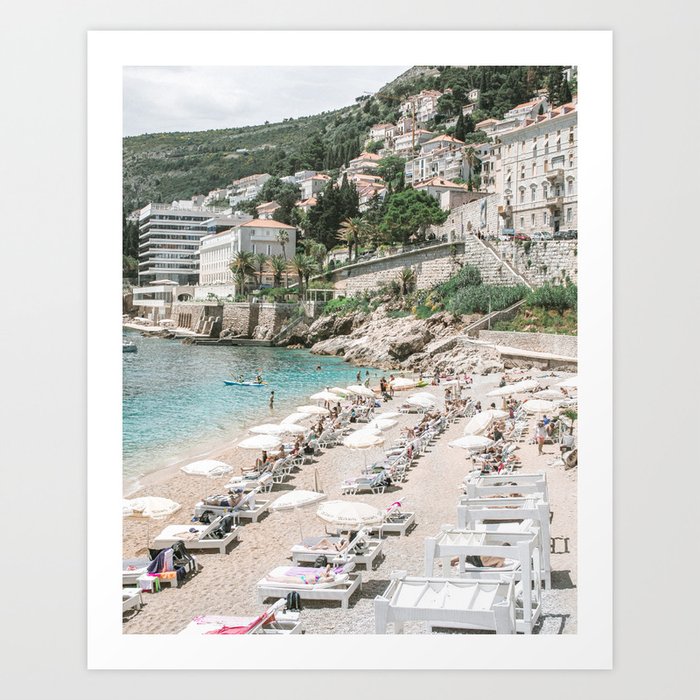This image portrays a stunning beachfront town where vibrant beach life meets lush, mountainous terrain. In the foreground, the sandy beach is dotted with rows of sun loungers and white umbrellas, some of which are elevated for sitting while others are flat for lounging. People populate the beach, basking under the umbrellas or enjoying the crystal-clear, blue ocean waters just 10 to 15 feet from the shore.

Behind the beach, a series of white brick buildings and modern glass structures ascend the side of a grassy, rocky mountain. The architecture blends seamlessly with the landscape, with roads winding upwards and connecting various hotels and houses. The mountainous backdrop covered in green vegetation enhances the scenic beauty, while the early morning sky, light blue with scattered white clouds, casts a serene ambiance over the entire scene. In the distance, the mountain's rocky structure contrasts beautifully with the lush greenery and the vibrant beach below.